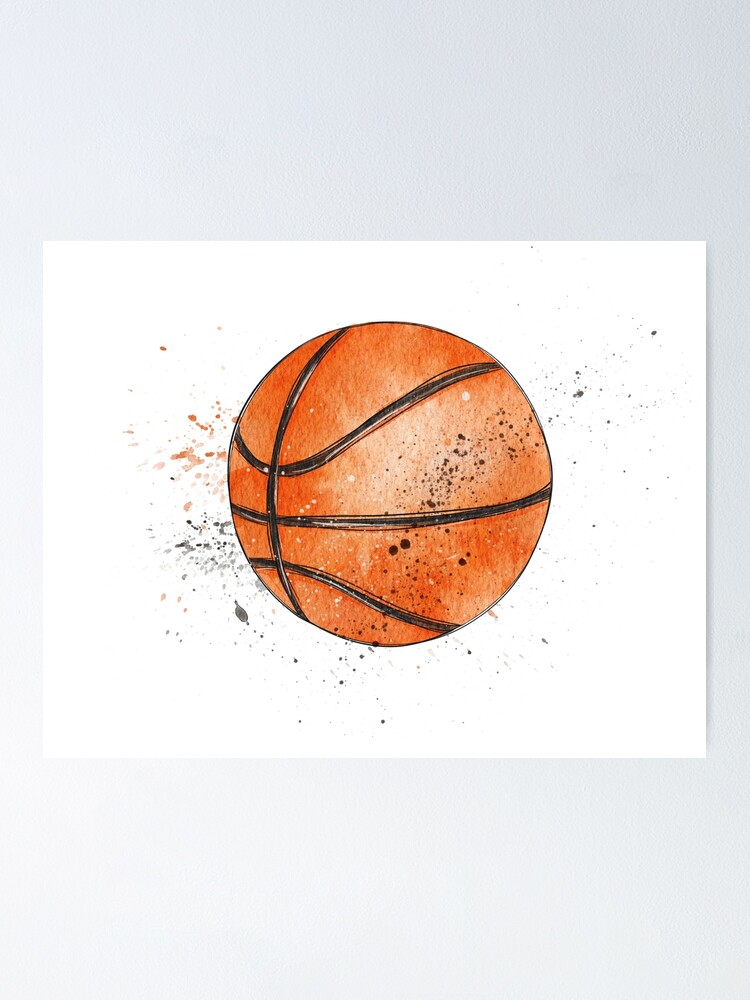This illustration, likely a piece of graphic design, depicts a classic round basketball set against a predominantly white background, giving the piece a minimalist aesthetic. The basketball itself is a vibrant orange with the characteristic black seams. The orange color varies in intensity, with lighter and darker areas creating a splotchy, watercolor-like effect. The artistic touch includes a splatter effect around the basketball, featuring drips and speckles of black, orange, and even pink, which add a dynamic sense of motion to the image. The basketball appears centrally placed on a white rectangle that is mounted on a grayish wall, enhancing its two-dimensional, yet vivid, presentation.